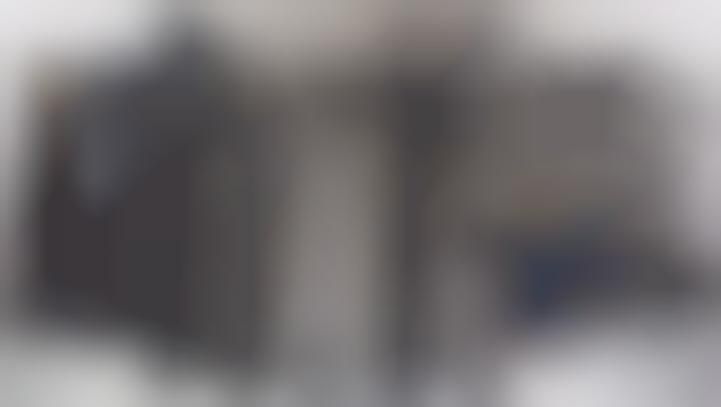The image appears to be extremely blurry, making it difficult to discern clear details. In the background, some shapes can just barely be made out, including what resembles parts of an accordion. On either side, there are black sections that could be the handles of the instrument, with white key-like parts on the right side of these black sections. There's a white part in the center that might be connecting the black sides, though it's very unclear. The overall color scheme of the image consists of dark blue, white, black, and some possible traces of faint pink on the right. The corners of the image seem lighter than the rest. The photograph is primarily characterized by an intense blurriness, with shadowy figures and splotches of varying shades of gray, black, and white, making it difficult to identify any definitive shapes or structures.